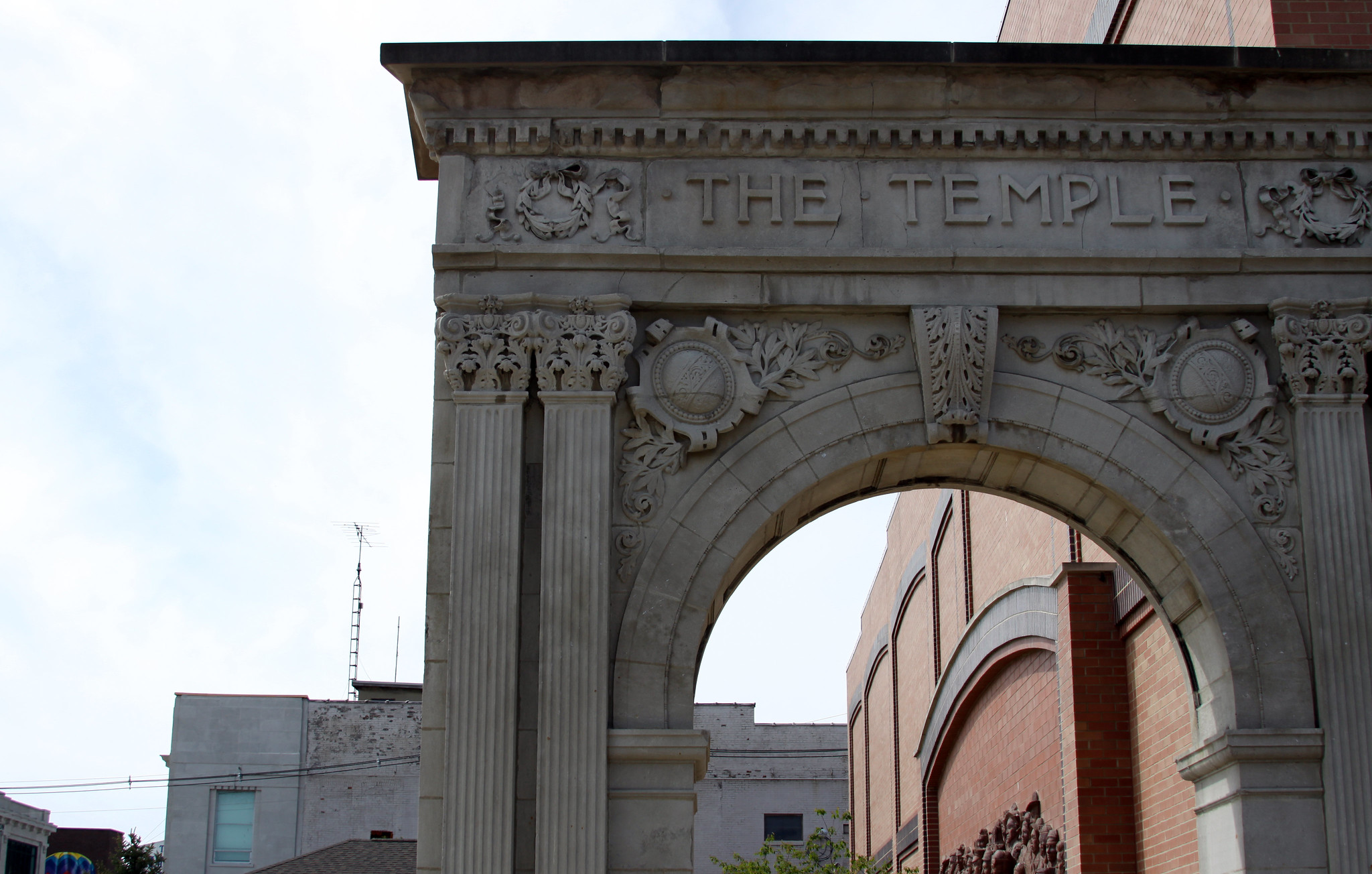The photograph captures an outdoor scene during daytime, showing a vintage, intricately designed archway that serves as the entrance to a temple. The archway, forged from gray stone, features elaborate carvings including two circular motifs adorned with leaf-like decorations. The words "The Temple" are engraved prominently at the top of the arch. The sky above is slightly cloudy with patches of blue showing through. In the mid-ground, just beyond the arch, is a brown, brick-and-mortar building situated to the right. Further back, to the left and center of the image, stands a gray-bricked building with a green-shaded window. Atop this building is a prominent radio antenna tower. The detailed and seemingly ancient architectural elements of the gate, paired with the urban backdrop of brick and gray buildings, contribute to the photograph’s overall historic and somewhat gaudy ambiance.